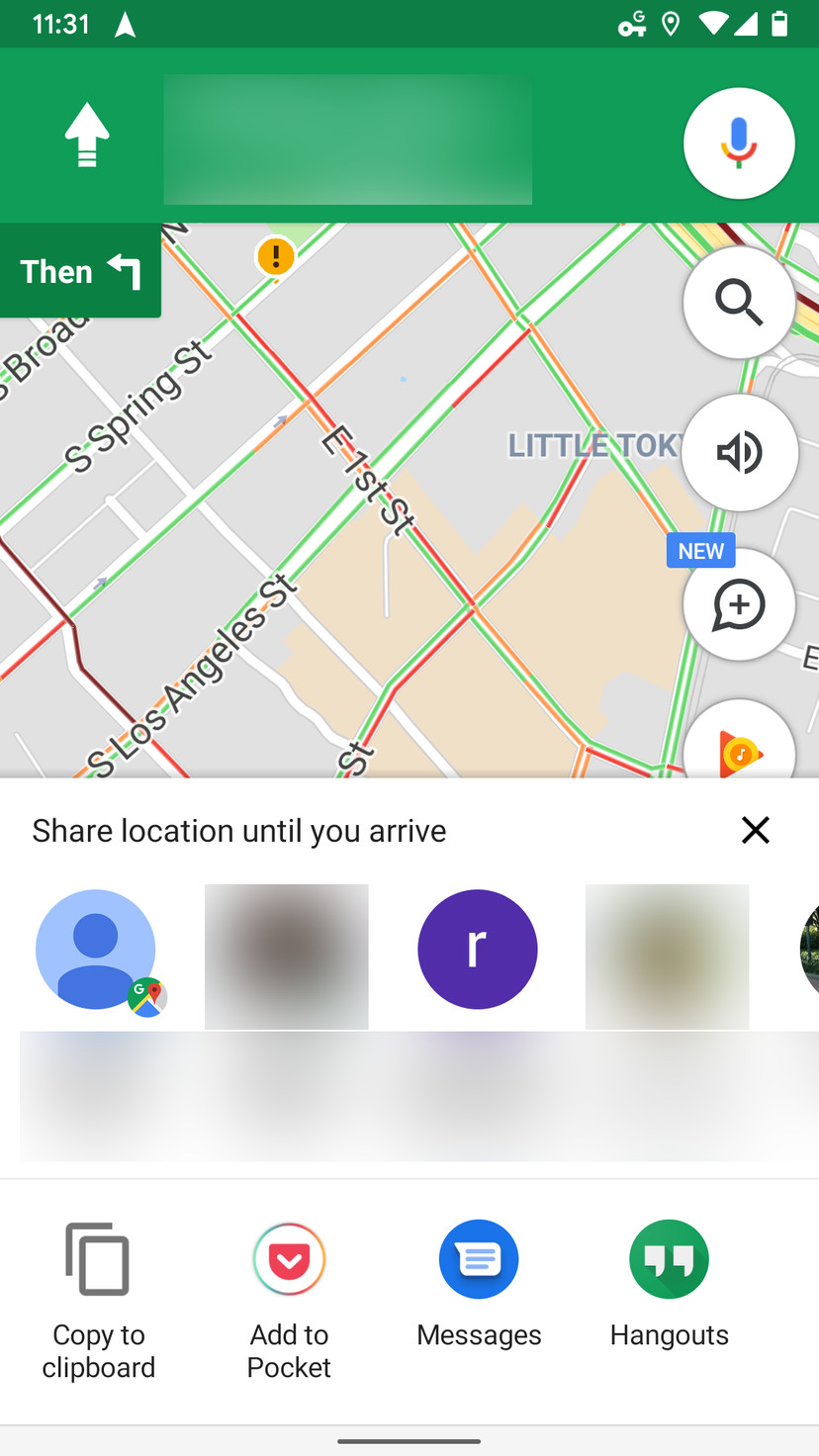The image is a screenshot of an Android device displaying Google Maps. The status bar at the top shows the time as 11:31, along with icons for location services, Wi-Fi signal, mobile network signal, and battery status. The main interface is dominated by the Google Maps application, characterized by its familiar green bar at the top.

The map itself is presented in grayscale, with white detailing for streets and green and red lines indicating different traffic conditions. The visual focus is on a particular area in Los Angeles, as evidenced by the mention of South Los Angeles Street. Key navigational features are evident: a microphone icon for voice navigation commands, a search symbol, a speaker icon, and a "+" symbol potentially for adding locations or waypoints. Additionally, a Google Music icon is noticeable, indicating an option to control playback within the app.

A prominent feature in the screenshot is a notification or option to "Share location until you arrive," listing different contacts with whom the location can be shared. Further interface elements include buttons for "Copy to clipboard," "Add to Pocket," "Messages," and "Hangouts," suggesting user-friendly options for sharing location details via various methods. The design employs a white background for buttons and options, contrasting against the gray map and the green navigation bar.

An arrow on the map hints at a direction for the current route, advising when and where to turn, but specific details are blurred to maintain privacy, ensuring no personal information is disclosed.